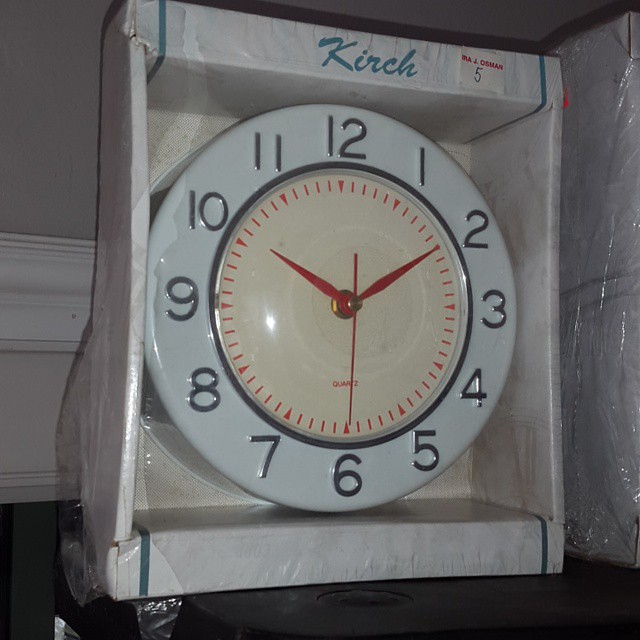The image depicts a wall clock still encased in its original packaging, placed on a dark-colored floor. The floor is accentuated by a white rail running along the base molding, and the adjacent wall is painted a medium shade of gray. The clock appears to be made of plastic, characterized by a large white frame encircling the clock face. The face itself is a yellowish white, adorned with simple black numerals from 1 to 12. Time markings are in red, and the hour, minute, and second hands share the same red hue. The clock operates with a quartz movement and is encased in a white cardboard box with a cellophane cover. The brand name "Kirch" is prominently stamped at the top of the box. It was purchased from Ira J. Osman and is identified as number 5.